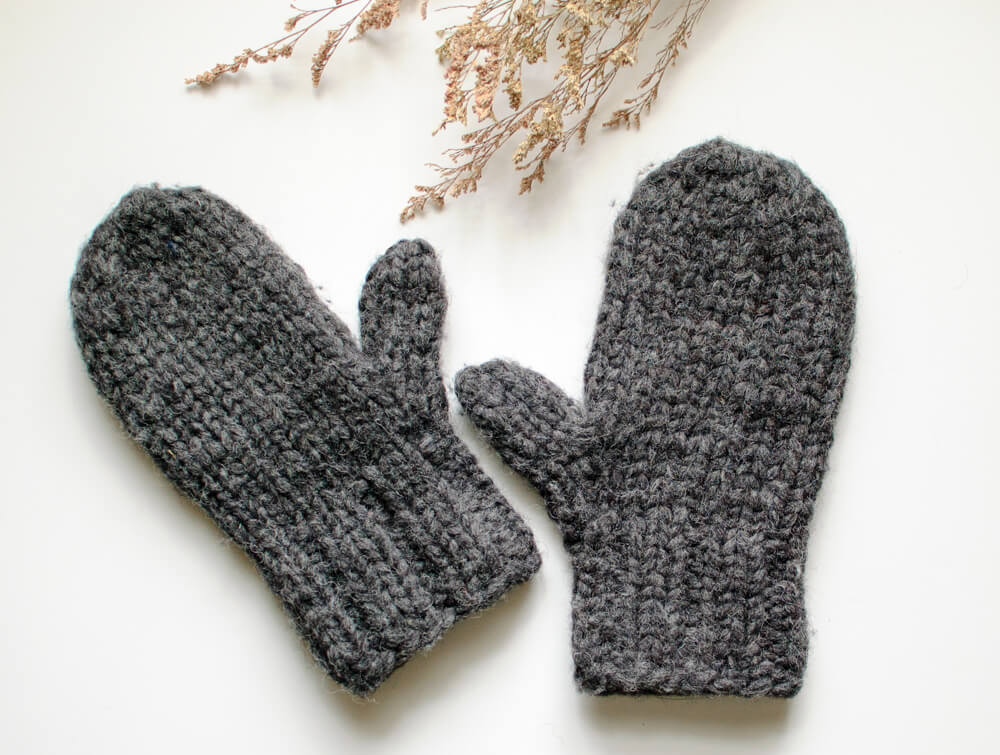This is a detailed image depicting a pair of gray, knitted mittens made from yarn, possibly wool, and designed to cover the wrist. They feature a thumb slot and a single compartment for the rest of the fingers. Both mittens are positioned on a white surface, with the left mitten laying diagonally from the upper left corner to the bottom center of the image, while the right mitten is placed vertically with the top of the fingers facing upwards. Above the mittens, in the top middle section of the frame, are some small, dried brown leaves or stems that add an accent to the composition. This landscape-oriented photo appears to be an e-commerce display, possibly showcasing women's mittens, and contains no text or additional imagery.